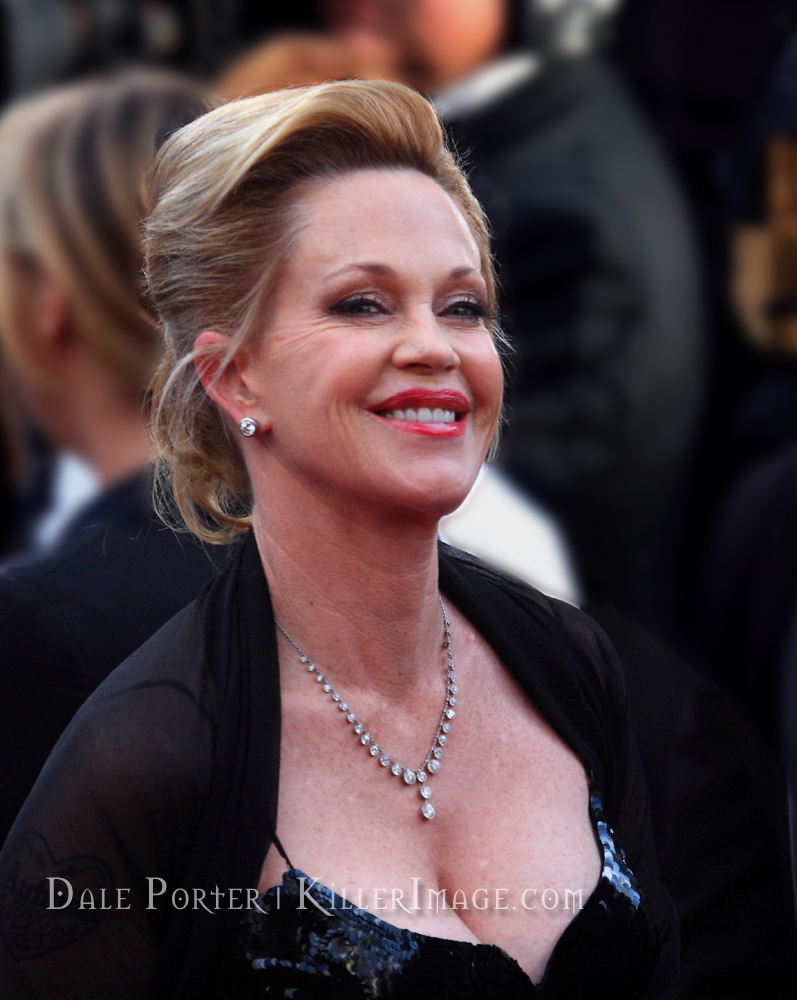This photograph captures a famous woman named Melanie, who is smiling warmly at the camera. Melanie is dressed elegantly in a black strapless, sequined dress, complemented by a sheer black shawl draped over her shoulders. Her ensemble is accentuated by a stunning diamond necklace that rests over her chest and adds a touch of sparkle. She is also wearing diamond stud earrings. Melanie's professionally styled blonde hair is pulled back, showcasing her radiant face adorned with orange lipstick. The photograph, which only shows her from the chest up, also has text at the bottom indicating "Dale Porter, KillerImage.com." The blurred figures in the background suggest that the photo was taken at a glamorous event, likely an award show or similar black-tie occasion.